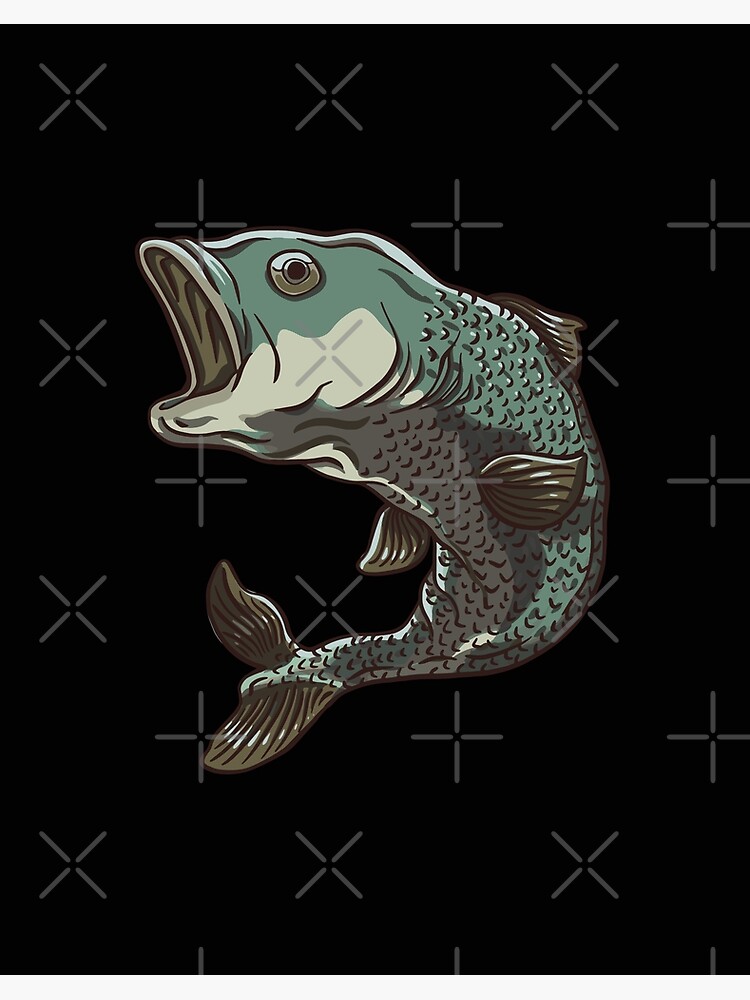The image depicts a computer-generated blue and grayish bass fish against a stark black background. The fish is shown with its mouth wide open, as if gasping for air, facing left in profile. The background features an array of gray symbols, predominantly X's and plus signs, arranged in rows that appear to float above and behind the fish, giving a watermarked effect. The fish showcases detailed scales and fins—its body is primarily blue with light gray on the bottom and an off-white or beige around the mouth area. The fish has a noticeable black eye, capturing a sense of depth and realism despite its digital rendering. The fins along its tail, sides, and top are distinct, adding to the intricacy of the overall depiction.